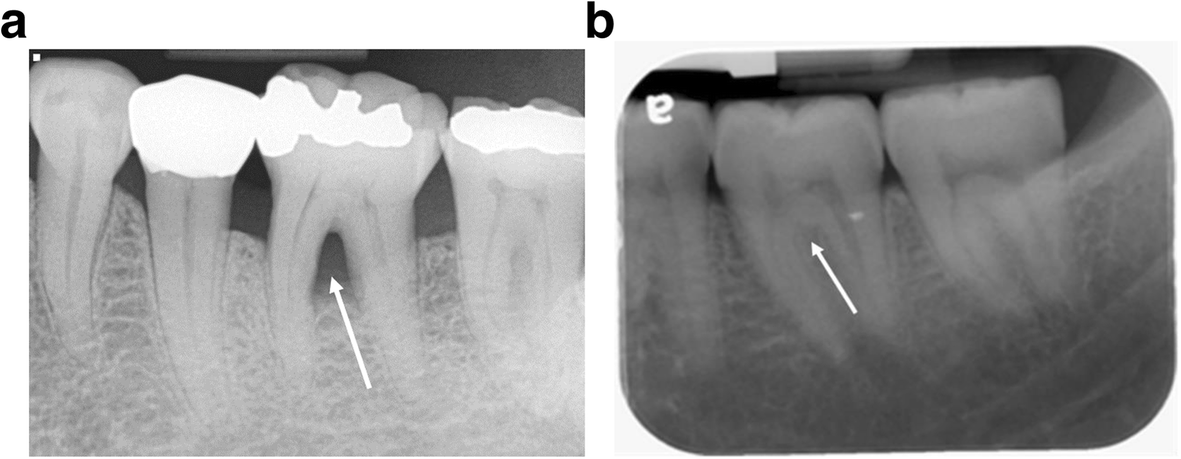The provided image consists of two black-and-white x-ray photos labeled A and B, each displaying sections of a person's teeth. The x-ray labeled A, located on the left, is slightly lighter, showcasing four teeth with visible crowns and cavity fillings on the molars. There is a white arrow pointing to a dark area indicative of a cavity at the root of the molar. In contrast, the x-ray labeled B on the right is darker and captures three teeth, with a white arrow similarly pointing to the root of the middle tooth, suggesting the presence of a cavity. The images reveal the roots and gum line, highlighting the affected areas with clear white arrows for detailed dental examination.